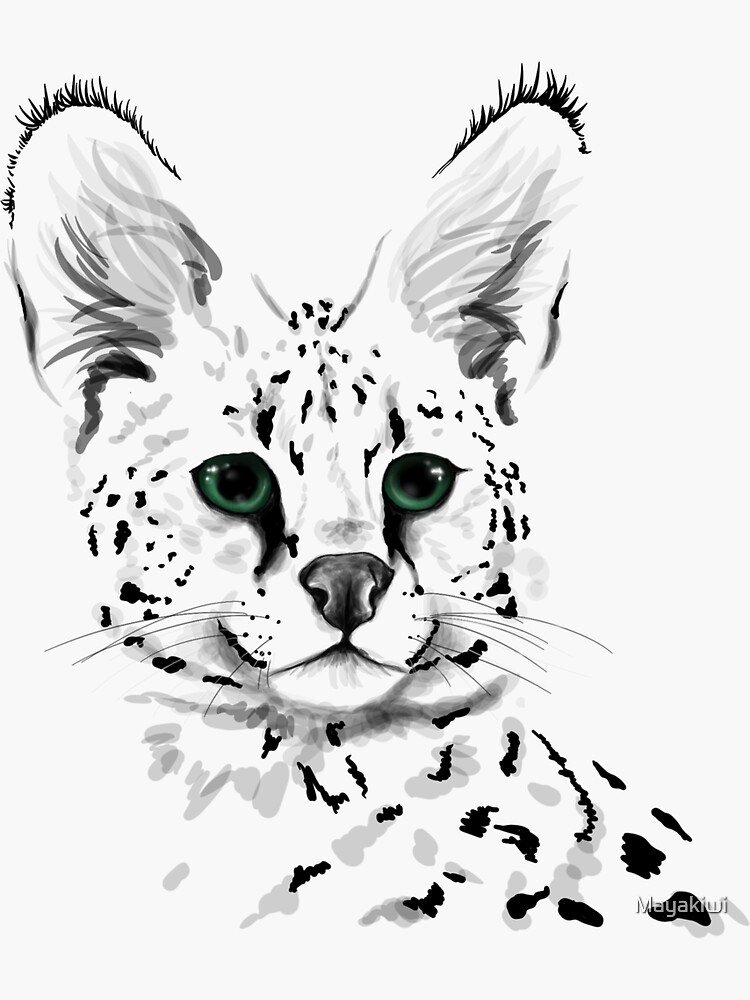This is a watercolor painting of a wild lynx, characterized by its large, pointed ears adorned with black hair tips and a distinctive white coat patterned with gray and black spots. The animal is depicted facing forward but gazing slightly to the viewer's right. The lynx’s head is the focal point, showcasing detailed features including an intricate nose, finely rendered muzzle, and soft emerald green eyes with dark pupils. The painting lacks any background, enhancing the contrast against the white paper. Transparent text at the bottom right reads "Maya Kiwi," completing the artist's signature.